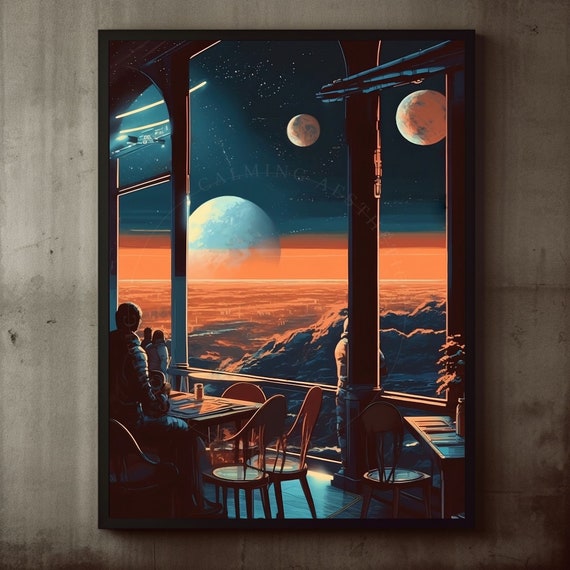The image depicts a futuristic-themed painting hung on a gray wall with a brown border that mimics the window separations. The painting portrays a high-in-the-sky restaurant or observation deck with large windows overlooking an otherworldly, outer space scene. Inside the restaurant, wooden tables and stools are occupied by silhouetted figures, possibly including a bartender. The background of the painting features a dark green and black outer space sky adorned with stars. Prominently, three planets are visible: a smaller blue one in the center, a larger orange-hued one to the right, and a partially seen large blue planet enveloped in an orange haze to the left. Below these celestial bodies are rocky formations in shades of orange and black. Overall, this oil painting creates a stunning and imaginative vista of people dining while gazing at the vastness of space.